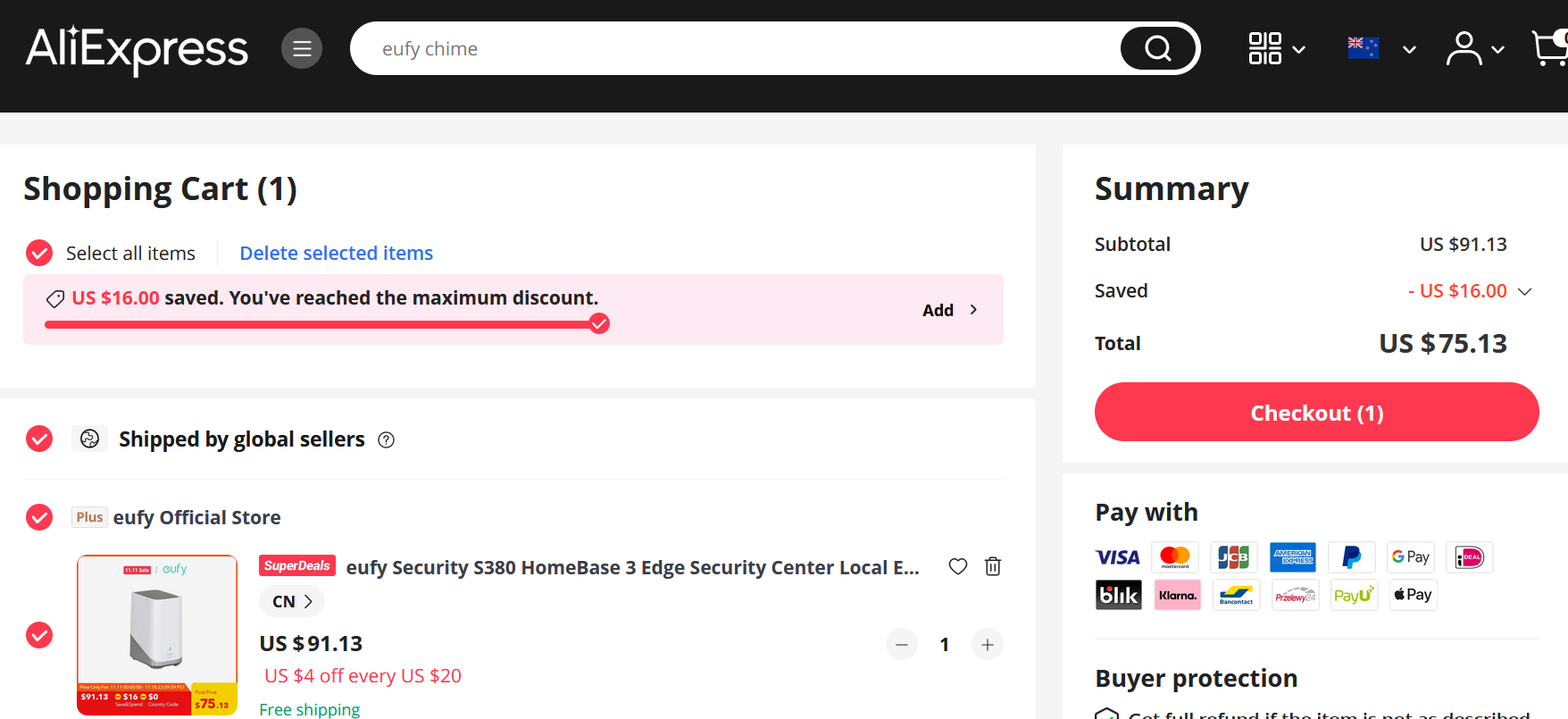The image depicts a shopping cart page from the AliExpress website. The screenshot shows a single item in the cart: the U5 Security S380 Homebase 3 Edge Security Center, priced at $91.13. Despite the item's value, the checkout total is displayed as $5.13, possibly due to discounts or vouchers applied. 

At the top of the page, there is a visible search field allowing users to look for additional products. The AliExpress logo is prominently positioned at the top left corner of the screen. The color palette of the page includes tones of black, red, white, and blue, which are typical of the AliExpress site design. Various payment options are listed under the checkout total, including Visa, MasterCard, Blink, Klammer, PrizeWheel, Google Pay, PayPal, and Apple Pay, offering a range of choices for the buyer to finalize their purchase.